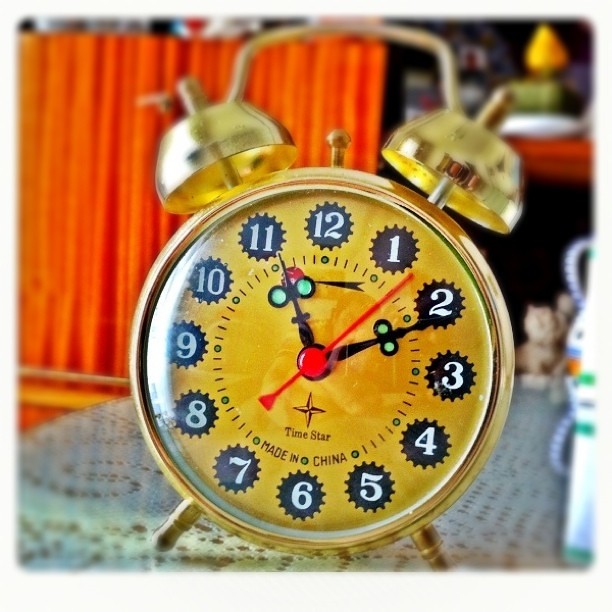This square, color photograph, framed by rounded and blurred edges, presents a charming, old-fashioned alarm clock standing on a table. The background features a faint, sharp white strip and orange curtains. This gold-colored clock is of the traditional design with two bells on top, connected by a small metal piece. The face displays plain Arabic numerals in white, enclosed within black circles adorned with small dots resembling little black suns. The clock's hands are old-fashioned: the hour and minute hands are black, while the seconds hand is red. Additional green and black markings indicate 15-minute intervals. The time on the clock is set to 10 past 11. The brand "Time Star" is marked with a Southern Cross star symbol, and "Made in China" is inscribed beneath it. The clock rests on a white doily atop a table, its details standing out against the blurred, rustic orange background.